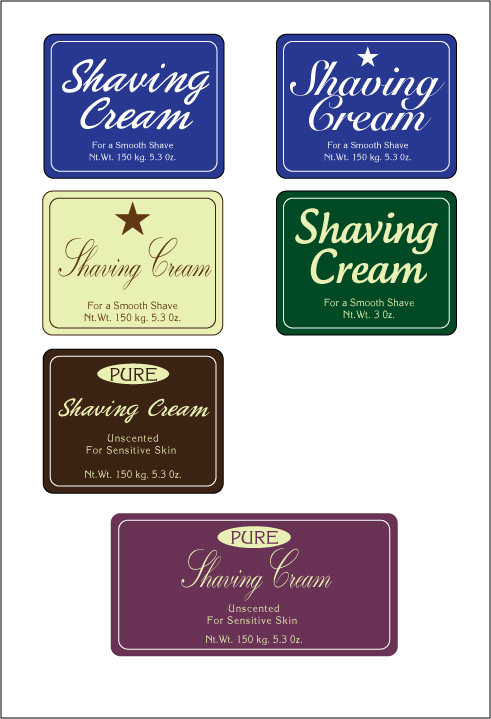This portrait-oriented, color image showcases six computer-generated designs for shaving cream labels, all featuring the same product details but varied in color, shape, and font. Each label prominently displays "shaving cream" with the tagline "for a smooth shave" and the net weight indicated as "150 kg" or "5.3 oz" except for one variant. The designs are arranged in two columns with three rows.

- **Top Left:** A dark blue square with a thin white border enclosing a smaller square, featuring "shaving cream" in white cursive text. A white subtext reads "for a smooth shave, nt. wt. 150kg, 5.3 oz."
  
- **Top Right:** Similar to the top left but includes a white star above the text. The label is blue, with the same product details in a curving font: "shaving cream, for a smooth shave, nt. wt. 150kg, 5.3 oz."

- **Middle Left:** A cream-colored square bordered in dark brown with a brown star. The text in cursive reads "shaving cream, for a smooth shave, nt. wt. 150kg, 5.3 oz."

- **Middle Right:** A chocolate brown square with a thin white border and a tan circle in the center. Inside the circle, "pure" is written in brown. Below, it reads "shaving cream, unscented for sensitive skin, nt. wt. 150kg, 5.3 oz."

- **Bottom Left:** A rectangular purple design with a white rectangular inset. It features "pure" in tan within a purple circle and white text "shaving cream, unscented for sensitive skin, nt. wt. 150kg, 5.3 oz."

- **Bottom Right:** A dark green square with a white inset. The tan text reads "shaving cream, for a smooth shave," but with a different net weight of "3 oz."

Together, these labels represent variations in design elements such as shape, font, and color while maintaining consistent product information across different aesthetic treatments.